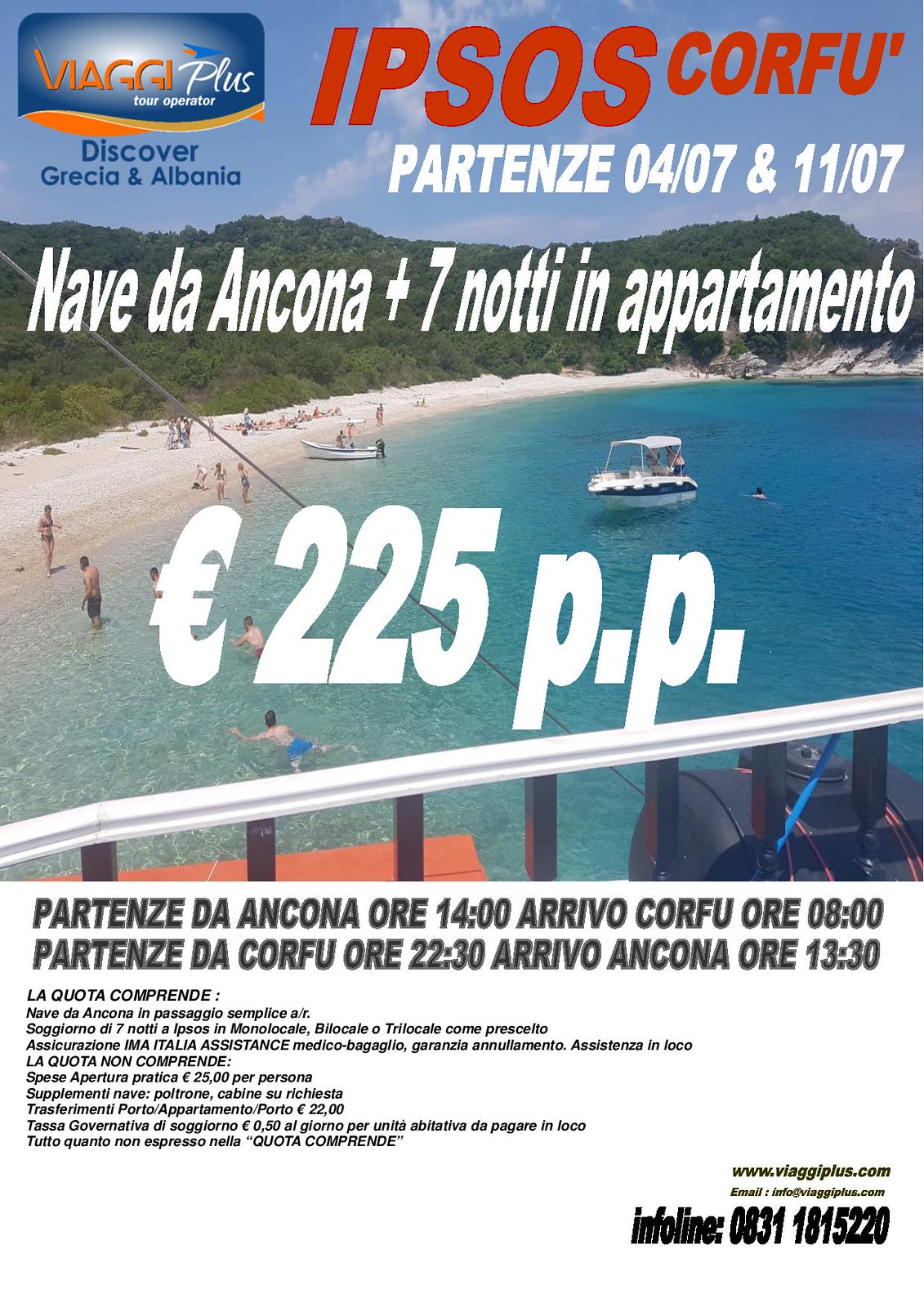The image is a detailed magazine cover for travel, emphasizing tours to Greece and Albania. At the top left, a blue banner reads "VIAGGI Plus Tour Operator," with "Discover Greece and Albania" below. The backdrop showcases a stunning coastal scene with a vibrant blue sky, green-clad mountains, and a pristine white sand beach fronting clear blue waters. Two boats are seen heading towards the shore where people are enjoying the beach and the water. The viewpoint is slightly elevated, possibly from a boat or a building.

Prominent text includes the large red bold print "IPSOS" at the top, with "CORFU" in smaller red print beneath it. Below, "PARTENZE 04/07 & 11/07" is written in white, followed by "NAVE DA Ancona + 7 notti in appartamento." Additionally, a significant symbol is featured alongside "225 P.P." Below this, text in Greek and/or Spanish is partially visible, suggesting the location’s authentic allure. The bottom section includes contact information: "info line: 0831 1815220" and a darker, bolder "www.viaggiplus.com", with an unclear email address nearby.